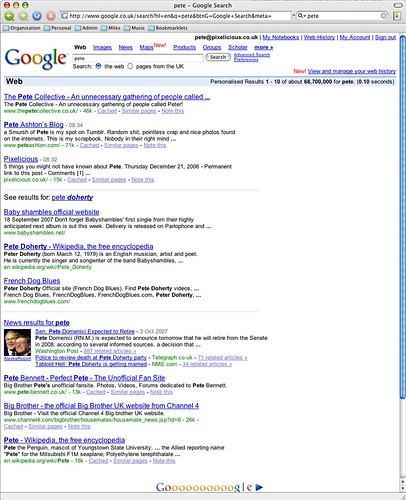The image appears to be a screenshot of a Google search results page displayed on someone's computer screen. At the very top, the interface features a gray toolbar labeled "Google search." Centered in a white background is the prominent Google logo, indicating that the user has conducted a search. Below the logo, a list of search results is visible.

The first search result appears to be titled "The Pete Collective and Unnecessary Gathering of People Called," and is followed by a link to "Pete Ashton's blog." The next result seems to be related to "Pixalicious," and includes a suggestion to "see results for Pete Doherty." 

Further results include "Baby Shambles official website," an entry for "Pete Doherty" on Wikipedia, and a link titled "French Dog Blues." There is also a section for news results, which mentions an article related to "Senator Pete Doherty expected to..." although the text is too small to read in detail.

Subsequent results feature "Pete Bennett," described as "Perfect Pete, the unofficial fan site," and a link to the "official Big Brother UK website" on Channel 4. Finally, another Wikipedia entry for "Pete" is included.

Overall, the screenshot captures a typical Google search results page focused on various individuals named Pete, with several references to notable personalities and their associated websites or fan pages.